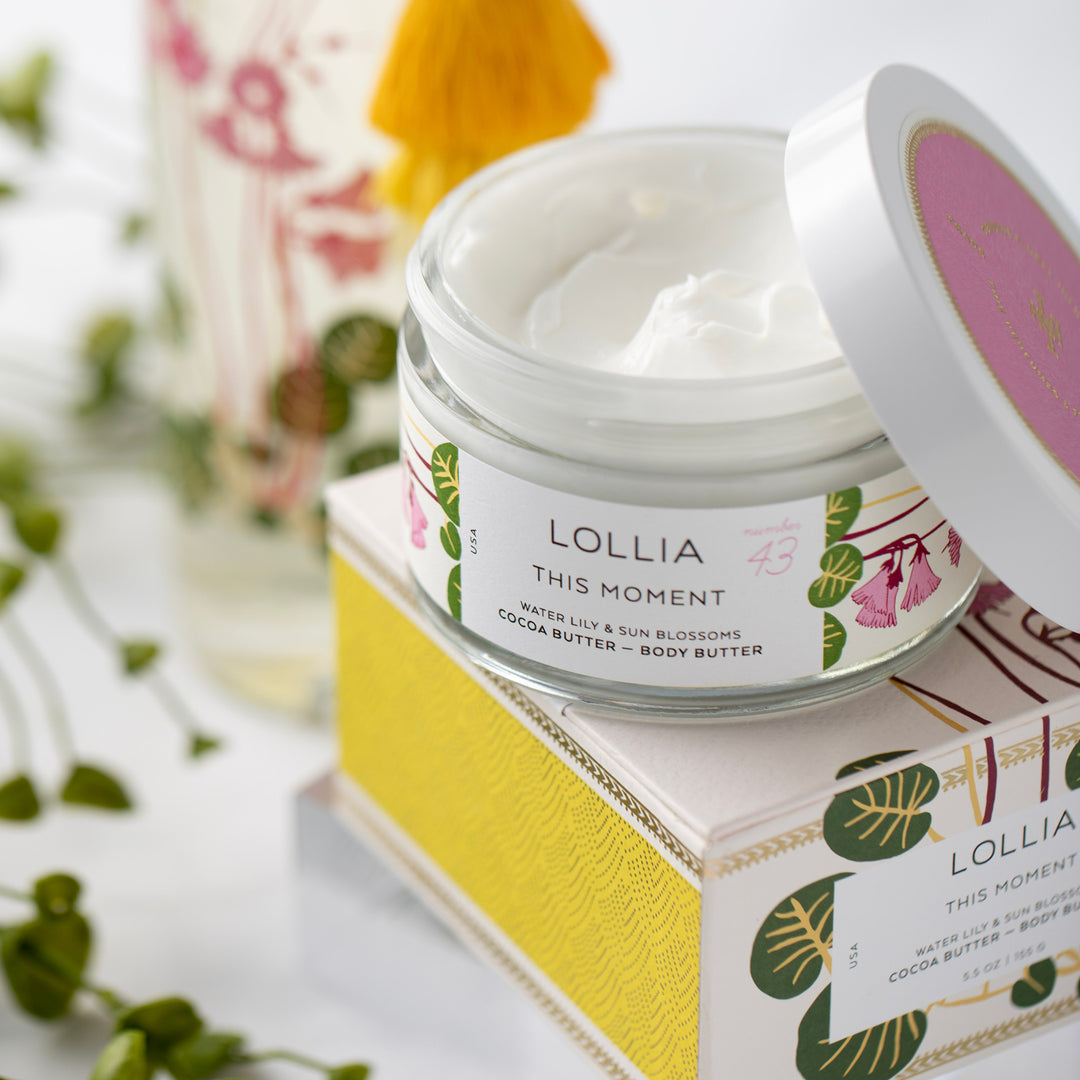This image showcases a beautifully presented product, likely intended for an advertisement. The focal point is a jar of body butter, identified by the label as "Lollia." The jar displays multiple inscriptions, including "this moment," "water lily and sun blossoms," and "cocoa butter body butter." The white jar features decorative elements of pink flowers and heart-shaped green leaves. The jar is placed atop a matching box, which shares the same floral and leaf motif and is detailed with a yellow ribbon. The jar's cap, also white, rests beside it, revealing the thick, white cream inside. The background enhances the presentation with blurred green leaves and flowers, creating an inviting, nature-inspired ambiance.